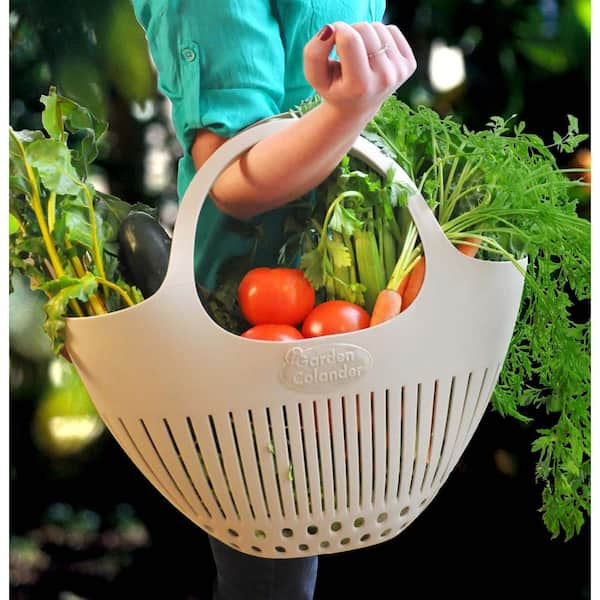A photograph captures a woman from the torso down to her knees, holding a white garden colander basket draped over her bent arm. The basket bears the text "garden colander" and features lines and circular cutouts for drainage. It is filled with freshly harvested garden produce, including tomatoes, carrots with stems, celery, an eggplant, a large zucchini, and an unidentifiable leafy green vegetable. She is wearing a teal blue button-up blouse with sleeves rolled up past her elbows and denim jeans. Her hand, positioned upward in the basket's loop, showcases maroon nail polish on the thumb and a ring on the middle finger. The background is blurred, hinting at a combination of green foliage, sunlight, and dark areas, likely indicating the photo was taken in natural daylight but with a shallow depth of field.